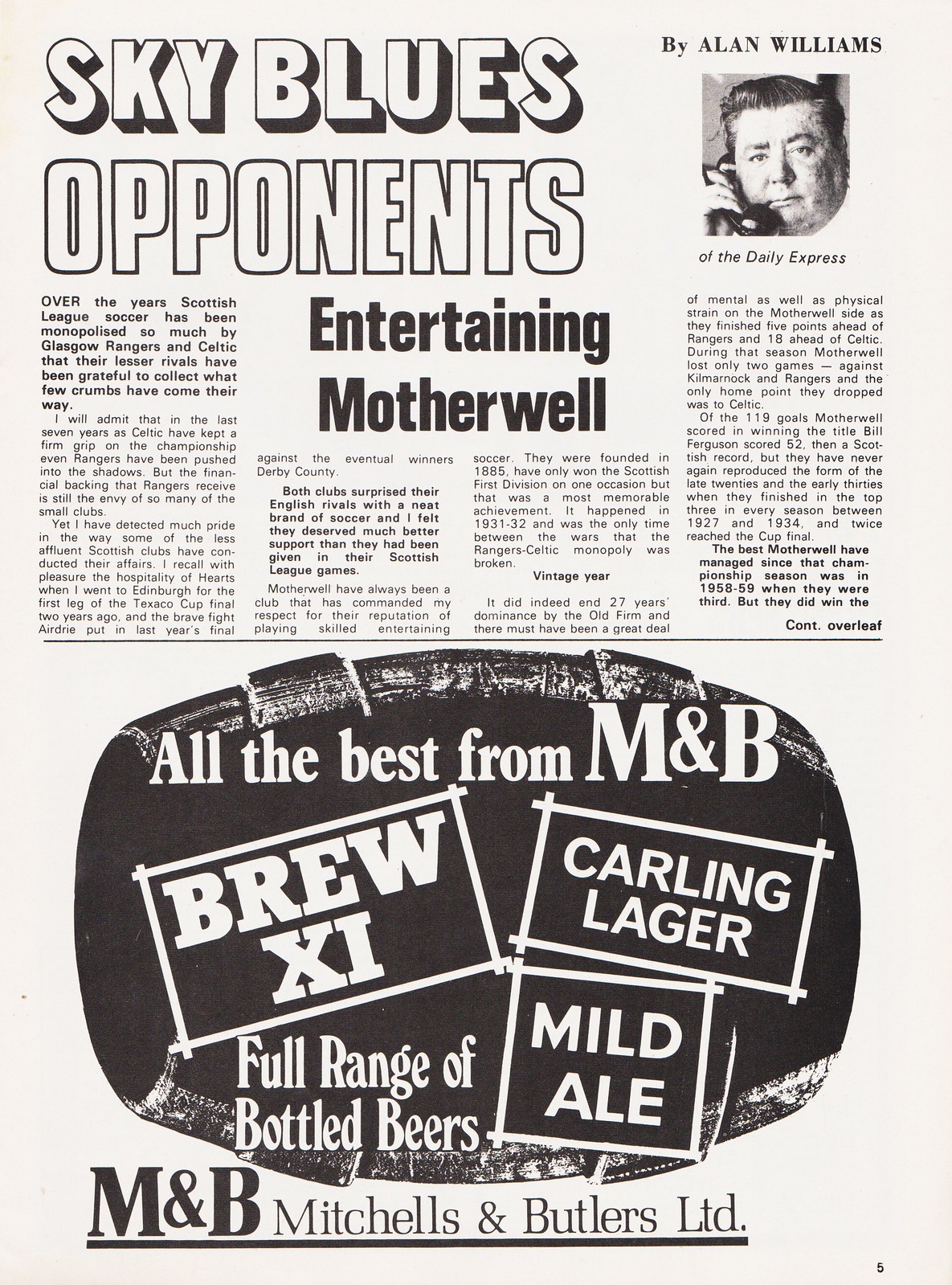This detailed black-and-white page, taken from an official game day program, merges sports journalism and vintage advertising. The page, which is in portrait orientation, is divided into two main sections. The top half features an article titled "Sky Blues Opponents" with a secondary headline, "Entertaining Motherwell," centered beneath it. This section contains four columns of text that delve into the dominance of Glasgow Rangers and Celtic in Scottish league soccer. At the top right, there is a small black-and-white profile photograph of a man talking on the phone, accompanied by the byline, "By Alan Williams of the Daily Express." The article, which appears to be continued on the following page, offers extensive insights over several paragraphs.

The bottom half of the page features a vintage-style advertisement for Mitchell's and Butler's Limited. This ad is dominated by an illustration of a barrel lying on its side with text overlaying it. The heading states, "All the Best from M&B," followed by a description of Brew XI, Carling Lager, Mild Ale, and a full range of bottled beers. The text is creatively positioned in white within black rectangles at various angles, matching the nostalgic aesthetic of a mid-20th-century print publication. The entire layout, from the sports analysis to the promotional content, captures a retro charm characteristic of classic game day programs.